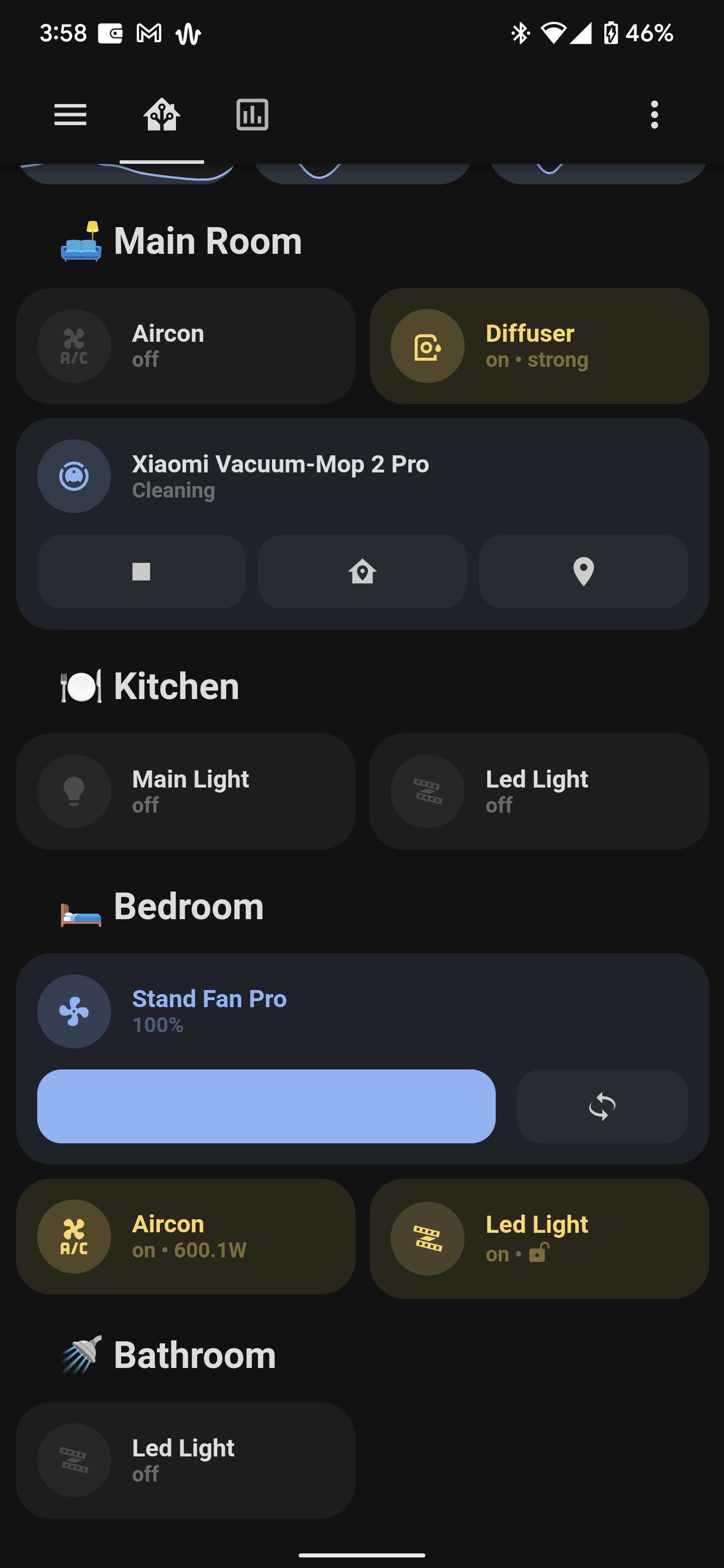Vertical screenshot of a smartphone interface with a black background. At the top, the status bar displays the time "3:58" in white, along with various icons including a rectangular white icon, the Google Mail (M) icon, an upside-down M (W) icon, Bluetooth, Wi-Fi, cell reception, and a battery indicator showing 46% remaining. 

Below the status bar, a navigation bar features a hamburger menu icon, a home icon, a graph icon, and three vertical dots aligned to the right.

Directly under this bar, the screen shows sections labeled "Main Room," "Air Con," and "Diffuser." The text "XISOMI XIAOMI vacuum-mop 2 pro" follows, indicating the device's status as "Cleaning" with controls labeled "Stop," "Home," and "Location."

Further down, additional sections list various smart home devices including:
- "Kitchen" followed by "Main Light" and "LED Light" to the right.
- "Bedroom" with "Stand Fan Pro" below, accompanied by a light blue circular icon featuring a blue fan symbol and a blue horizontal button beneath it.
- "Air Con" highlighted in yellow, with an LED light indicator.
- "Bathroom" again featuring "LED Light" underneath.

The meticulous layout and iconography make it clear that the application is designed for managing multiple smart home devices, providing various interactive controls for each device displayed on the interface.